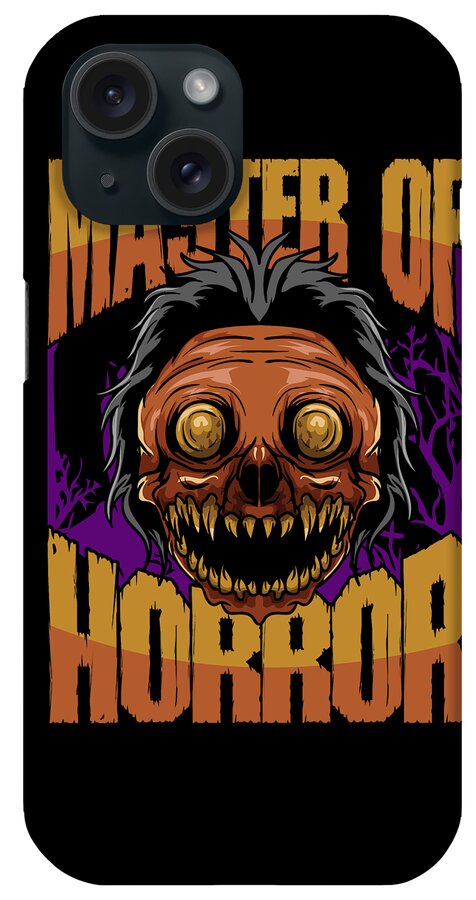The image is a detailed view of the back of a black iPhone case, designed for one of the newer models featuring a dual lens camera system. The case prominently displays the text "Master of Horror" in a gradient from yellow at the top to orange at the bottom. The phrase "Master of" is positioned at the top, while "Horror" is at the bottom.

Dominating the center of the case is a striking cartoon animation of a monstrous creature with an orange face, black wispy hair, and large, haunting yellow eyes without visible pupils. Its ghastly mouth is filled with jagged, long yellow teeth, and it has inflamed nostrils in place of a nose. Surrounding the creature's face are purple lines, contributing to the eerie color scheme that includes shades of yellow, orange, and purple, all set against the black background of the phone case. The design elements of the case are slightly obscured by the positioning of the camera lenses, yet the text and image remain largely legible.